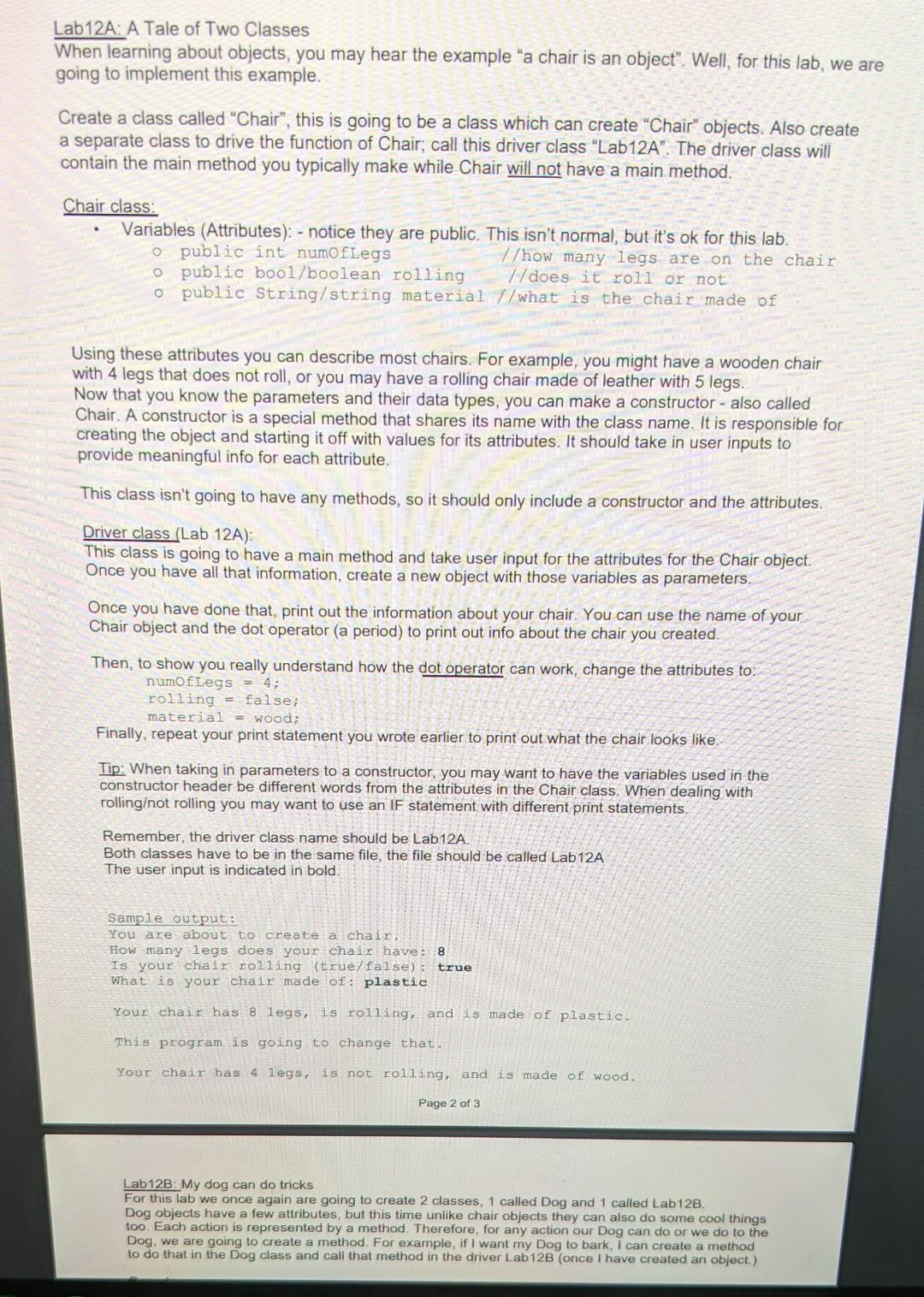**Caption:**

The image is a vertical rectangular piece of paper, likely white or cream-colored. At the top, the title reads "Lab 1-2-A: A Tale of Two Classes" in black font. The text below outlines instructions for a programming lab focused on understanding and creating classes in an object-oriented programming language.

The description begins with an introductory paragraph explaining the common example used to teach objects: "a chair is an object." For this lab, students are required to implement this example by creating a class named `Chair` that can generate chair objects, and a driver class named `Lab 1-2-A` to manage these objects. The driver class contains the main method while the `Chair` class does not.

The `Chair` class section, which is underlined, details its variable attributes—public for this exercise: the number of legs the chair has, whether it rolls or not, and the material of the chair. Although some of the writing is unclear, the right side mentions these specifics, while the left side remains unreadable.

The following paragraph explains how these attributes help describe various types of chairs, providing examples like a wooden chair with four legs that does not roll and a rolling chair made of leather with five legs.

Next, the explanation focuses on the constructor for the `Chair` class, a special method sharing the class name. This constructor sets initial values for the attributes using user inputs. Since the `Chair` class won't contain any methods, it only requires the constructor and attributes.

Moving on to the `Driver` class section, also underlined, it is explained that this class will have a main method to take user input for chair attributes, use these inputs to create a new chair object, and then print out the object's details. For proper function, the dot operator (underlined) is used to access and modify the chair's attributes, demonstrating comprehension of the concept by changing attributes and reprinting the updated chair details.

The text concludes with tips for ensuring clear variable names within the constructor to avoid confusion, suggesting different variable names from the attributes. It also mentions using conditional statements when dealing with rolling mechanisms, and stresses that both the `Chair` and `Lab 1-2-A` classes should be in the same file. Further specifics are too faint to read, but the foundation of the lab instructions is clear.